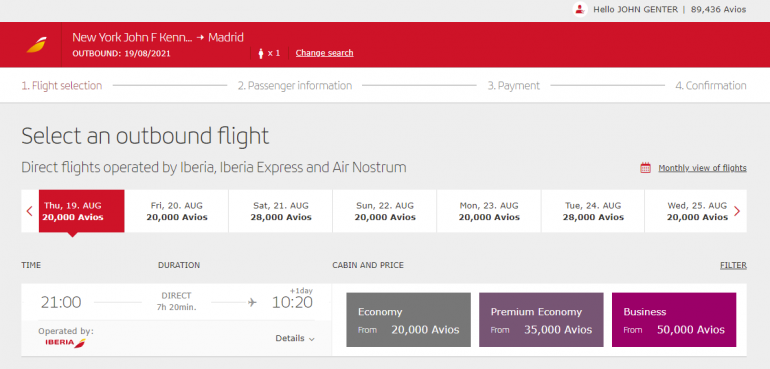Image Caption:

The screenshot depicts a flight booking website interface. At the very top is a red navigation bar featuring an airline logo with a swooping design. The flight details indicate a route from New York (John F. Kennedy Airport) to Madrid, accompanied by a right-pointing arrow. 

The outbound flight date is listed as August 19, 2021. Next to the date, an icon of a person indicates one traveler, with an adjacent option to change the search parameters.

Below this section, there is a step-by-step navigation process for booking: 
1. Flight Selection 
2. Passenger Information
3. Payment 
4. Confirmation

The primary instructions prompt the user to select an outbound flight. A list of available direct flights operated by Iberia, Iberia Express, and Air Nostrum is displayed, along with alternative dates spanning from Thursday, August 19 to Wednesday, August 25. 

Flight options are categorized by time, duration, cabin class (Economy, Premium Economy, and Business), and price, offering a comprehensive overview for travelers planning their journey.